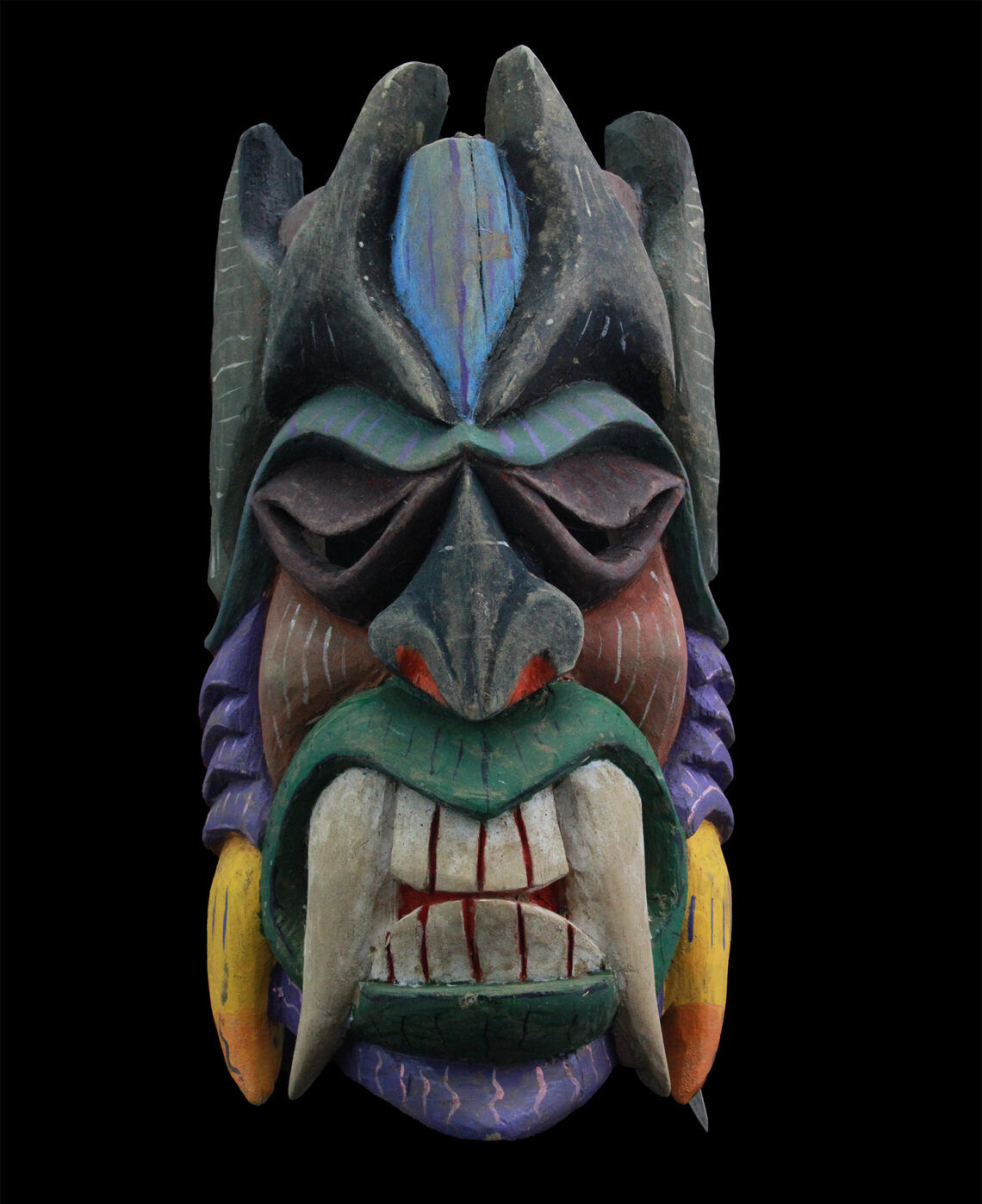The image features a detailed, colorful mask that appears to be an actual photo of a real, intricately carved mask, possibly inspired by Aztec, Mayan, or Polynesian cultures. The mask, set against a completely black background, is front-facing and vertically elongated with a prominent dark green, wide-open mouth displaying two large gray fangs and interspersed teeth. Surrounding the mouth is a green area, transitioning into red cheeks, and a purple chin with jagged stripes.

The mask exhibits vivid colors and complex patterns. Notably, it has a large nose with red or orange nostrils, and blue eyebrows above eyes that are purple and appear to be closed slits. The forehead features a blue section with an implied central jewel, flanked by black prongs or horns. The ears or earrings are purple, and large yellowish-orange rings are present at the bottom of the earrings. Contrasting brown cheeks add to the mask's striking and somewhat menacing appearance, giving it an overall impression of a demon-like face.

The intricate details, from the snorty, angry nose to the colorful, jagged patterns, contribute to the mask's elaborate and vivid depiction.